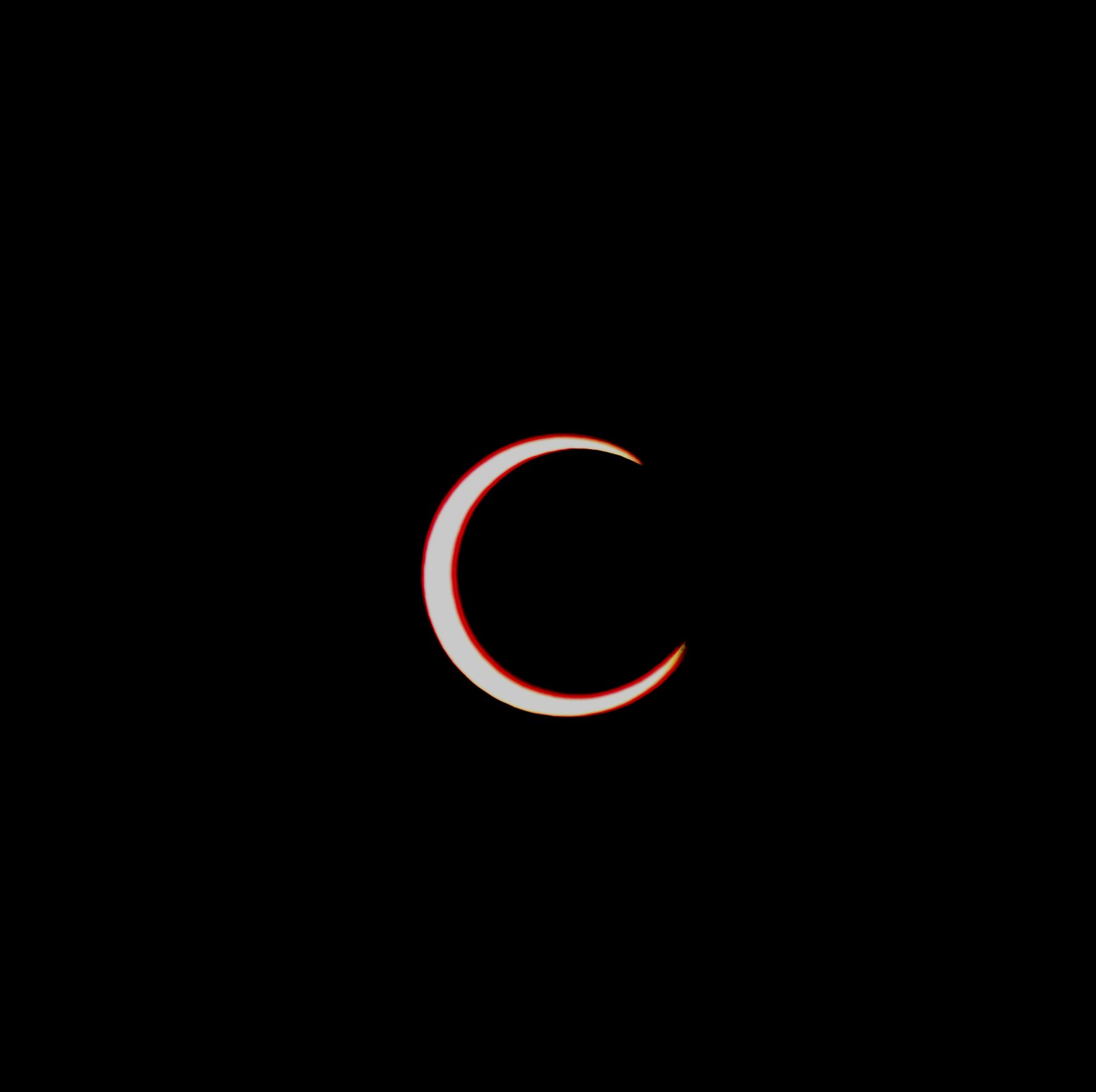The image features a digitally rendered crescent moon against a completely black background. The moon's crescent is sharp and thin, resembling a narrow C shape centered in the composition with its tips pointing slightly above the center line to the right. The design is highlighted with a striking red outline that becomes thicker and fades into a golden hue at certain points, particularly around the tips of the crescent. The middle section of the crescent's inner curve also features a prominent red outline that gradually blends into the blackness towards the top. This highly stylized and detailed depiction of the crescent moon, devoid of any text, suggests it may be a logo or a digital artwork rather than a real-life photograph, evoking the visual essence of a solar eclipse.